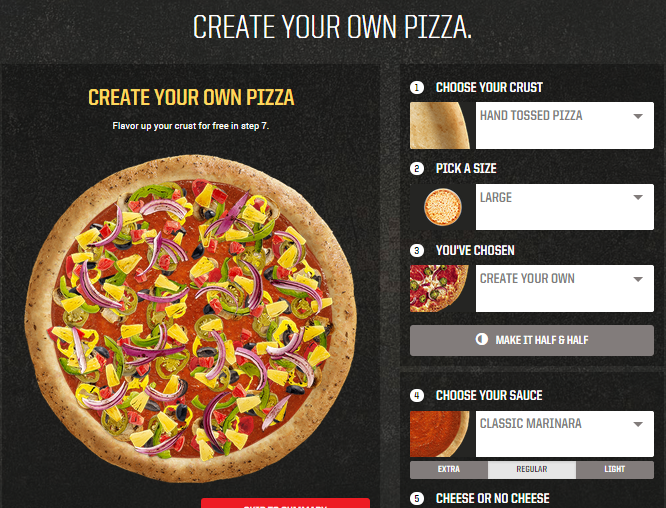Screenshot of a pizza ordering page with a black background and white text. At the top, in large print, it reads: "CREATE YOUR OWN PIZZA." The page is divided into two main sections. On the left side, it again says, "CREATE YOUR OWN PIZZA. Flavor up your crust for free in step 7" in all capitals.

Below this, there is an image of a round pizza, topped with various ingredients such as onions and peppers. Partially visible at the bottom of this section is a small portion of a red box, cut off by the page's edge.

On the right side, there are several sequential steps for customizing the pizza. 

1. "Choose your crust." This step is marked by a white circle with the number 1 inside. Below, it offers a "Hand Tossed Pizza" option with a pull-down arrow, accompanied by a close-up image of a pizza crust.
2. "Pick a size." This step displays a photo of a pizza and selection options for different sizes. Currently, the size is set to "Large," but a pull-down arrow indicates other available options.
3. "You've chosen." This step includes a close-up of part of a pizza. In the adjacent box, it says "Create Your Own" with an arrow beside it. There is also an option to make the pizza half-and-half.
4. "Choose your sauce." A close-up image of pizza with sauce is shown. In the menu next to it, "Classic Marinara" is selected.
5. "Cheese or no cheese," marked by a circle with the number 5. The rest of the page cuts off at this point.